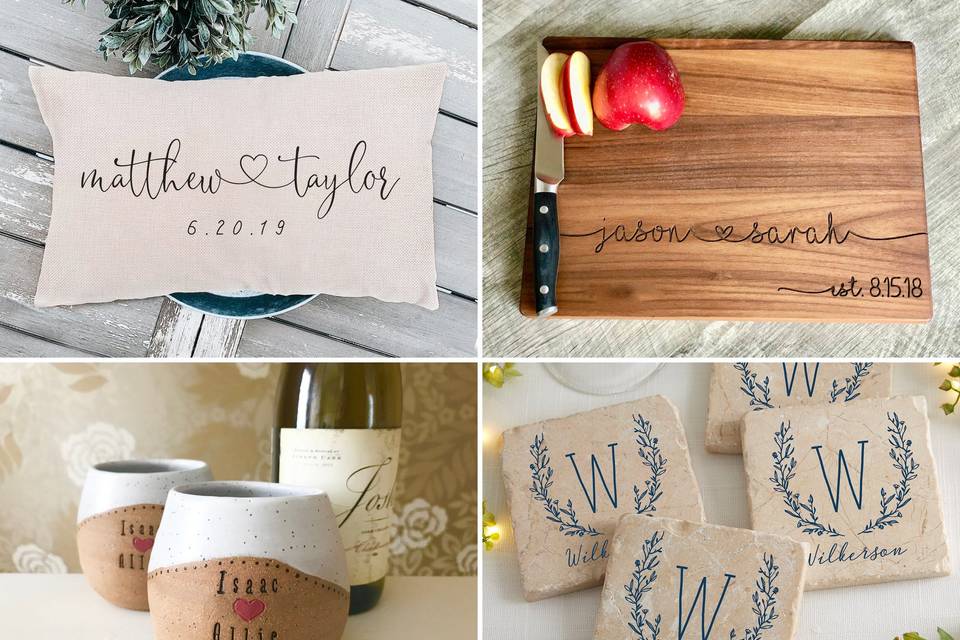The image comprises a horizontal rectangular arrangement of four smaller rectangles forming one large rectangle, with two on the top row and two on the bottom. In the upper left rectangle, there's a white card or possibly a pillow resting on a stainless steel or silver dish, bearing the inscription "Matthew Taylor" with a heart symbol and the date "6-2019." To its right, the upper right rectangle features a wooden cutting board inscribed with the names "Jason ♥ Sarah" and the date "8-15-18." This board displays a paring knife next to an apple that's partially sliced. In the bottom left rectangle, there's a wine bottle labeled "Josh Wine" flanked by two ceramic mugs. Lastly, the bottom right rectangle showcases white ceramic coasters with a large "W" in the center, likely indicating the initials "Wilkinson," surrounded by a wreath pattern. The overall composition appears to be promoting personalized home items.